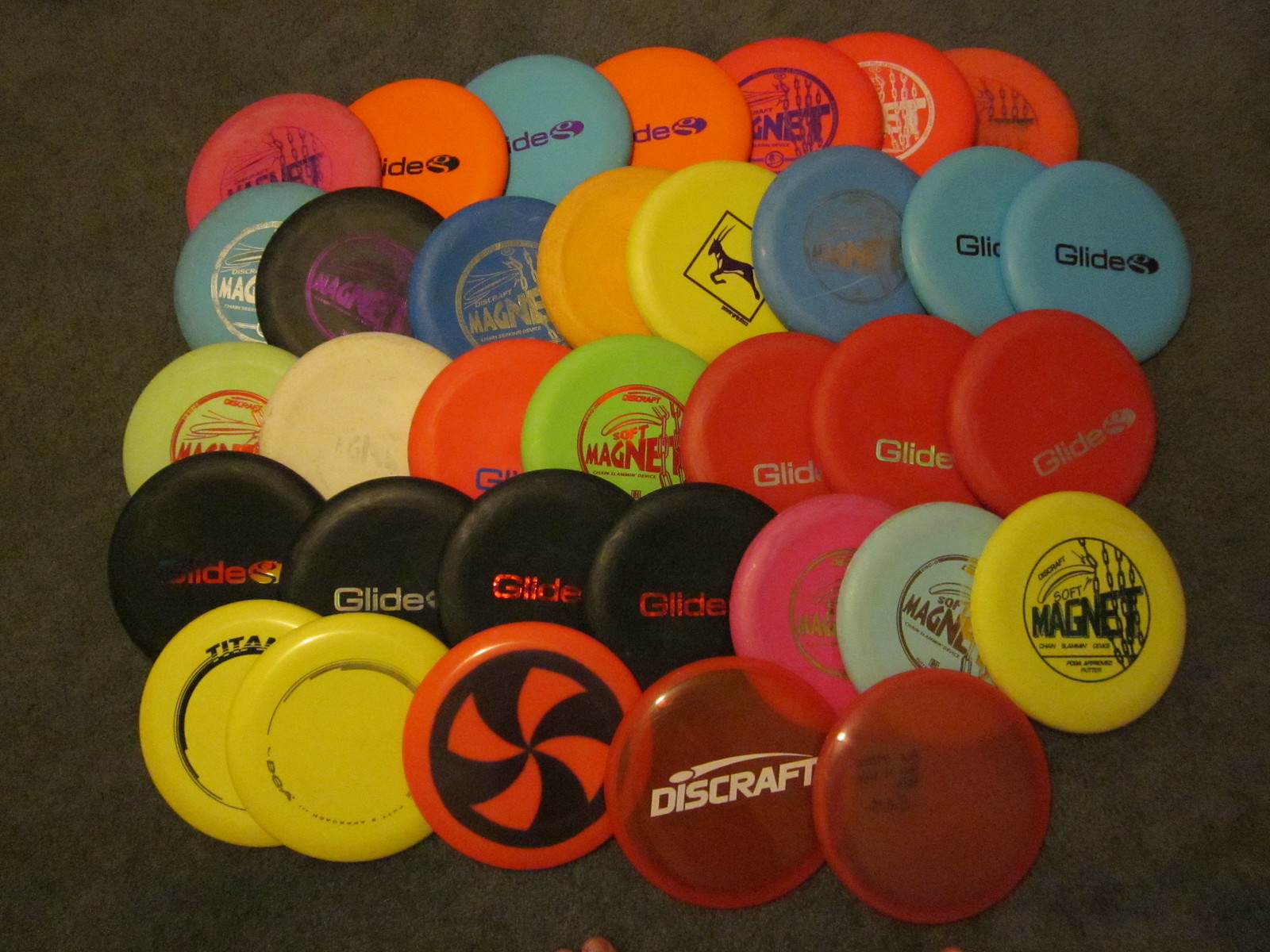The image is a close-up of approximately 30-35 miniature Frisbee-like discs, arranged in roughly five rows and up to seven columns, on a dark gray textured surface that resembles fine short-haired carpet or flooring. The discs are used in frisbee golf, featuring various colors such as yellow, black, orange, translucent orange, hot pink, dark pink, red, and blue. They display different logos and names, including brands like Discraft, Glide, Titan, DGA, and Soft Magnet. Some discs have unique designs, like a deer crossing sign. The arrangement is orderly but not perfectly uniform, showcasing the vibrant diversity of the collection.